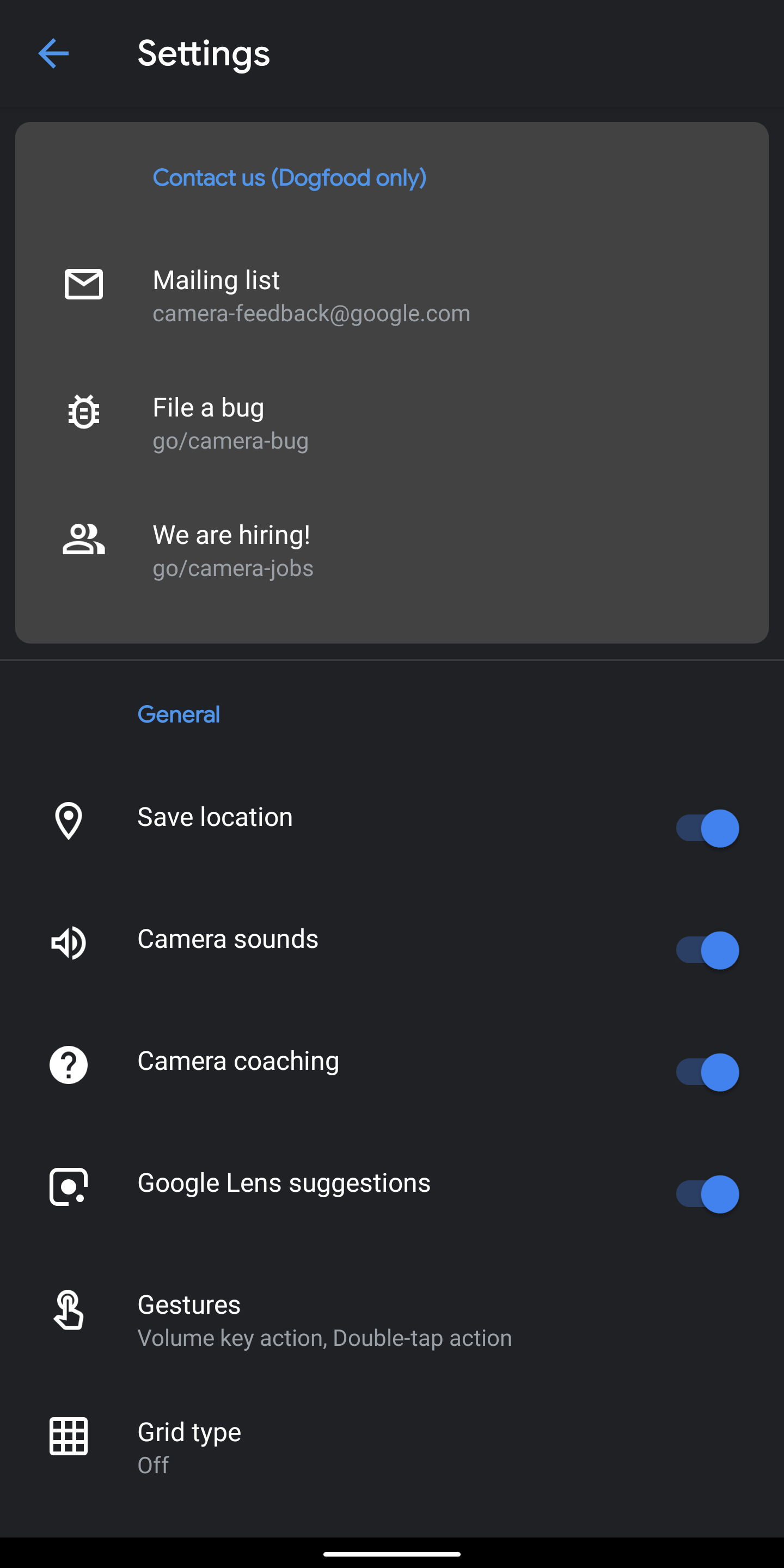The image depicts the settings page of a website displayed on an iPhone, featuring a sleek black background with white text and blue accents. At the top of the page, there is a blue arrow pointing left, accompanied by the text "Contact Us (dog food only)" in blue. Below this, "Mailing List" is written in white, alongside an envelope icon, followed by the email address "camera-feedback@google.com." The page also allows users to file a bug report via "Go/camera-bug" and shows a hiring link as "Go/camera-jobs."

The next section is labeled "General," continuing with the black background. It features various settings options including:
- "Save Location" with a white pin icon and a blue slider that can be toggled on.
- "Camera Sounds" with another blue slider for toggling.
- "Camera Coaching" also with a blue slider available for toggling.
- "Google Lens Suggestions" with a blue slider that is currently turned on.

Under the "Gestures" section, the page lists:
- "Volume Key Action"
- "Double-Tap Action"
- "Grid Type," which is noted as being off.

The design is minimalistic yet functional, offering concise and clear settings options for users.